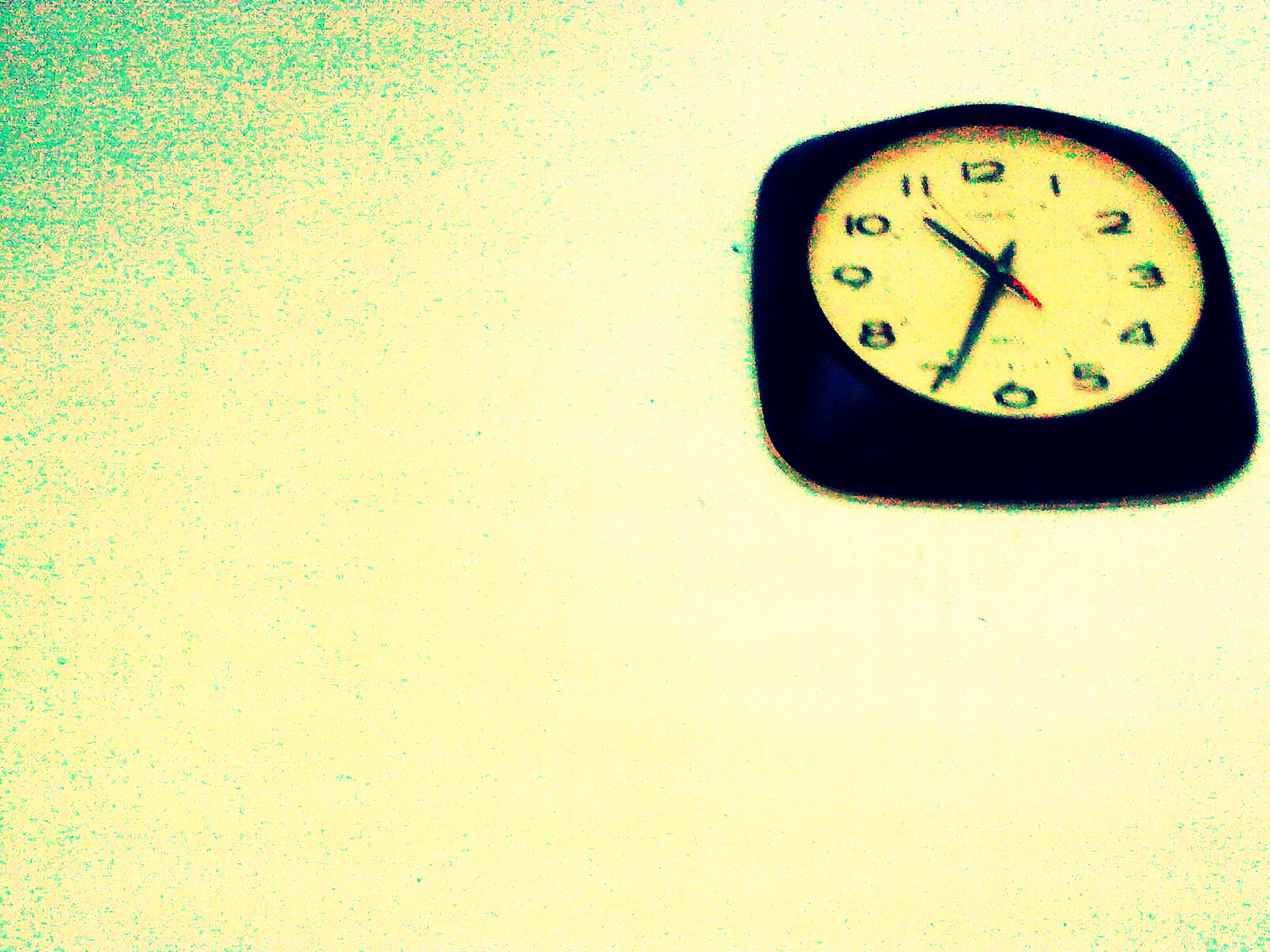The image depicts an off-center photograph of a wall-mounted clock. The photograph has an off-color tone, with a darker contrast background against a wall that seems to be either an eggshell white or a light yellow mustard color. A subtle tinge of light green permeates the top left corner of the image, adding to its vintage feel. The clock itself is positioned towards the top-right side of the photograph, framed in a black square. At its center is a circular clock face secured behind clear glass. The clock face is predominantly white, featuring bold black numbers ranging from 1 to 12. The time displayed is 10:35 p.m. and 55 seconds, indicated by sleek black hour and minute hands and a vibrant red second hand. Due to the off-center composition and lighting, the brand name of the clock remains unreadable.